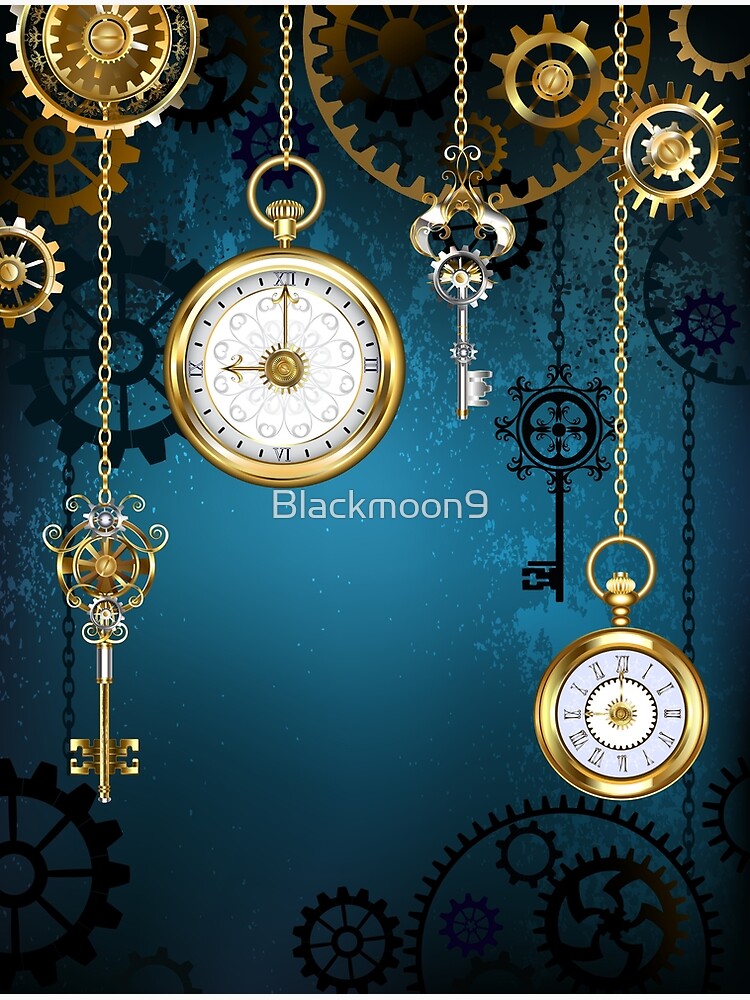The vertically oriented poster features a blue background adorned with intricate illustrations of gears, keys, and chains, evoking a steampunk aesthetic. Gold gears and individual black cogs and wheels are scattered throughout, enhancing the mechanical theme. Chains hang from the top, displaying an array of timepieces and keys. On the left side, a gold gear supports a chain from which a skeleton key dangles. To its right, a series of three chains descend from the top—each showcasing a different item: a pocket watch, another skeleton key, and another pocket watch, all in gold. Central to the design, just below a pocket watch, the name "Black Moon 9" is prominently written in white text. The pocket watches are noticeably set to nine o'clock, linking to the brand name. The overall composition suggests an advertisement for Black Moon 9, emphasizing their intricate, steampunk-inspired timepieces and accessories.